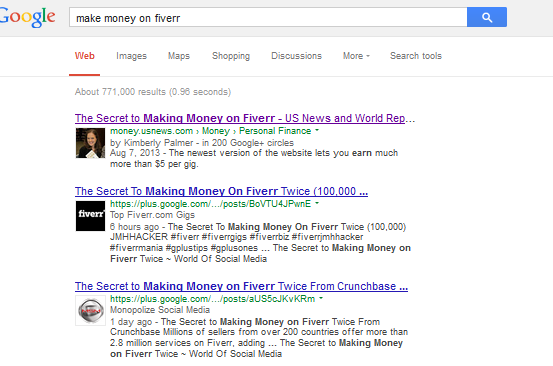A detailed caption could be:

"This is a screenshot of a Google search results page for the query 'make money on Fiverr.' The search bar at the top contains the typed query. Below the search bar, there are several tabs: 'Web,' 'Images,' 'Maps,' 'Shopping,' 'Discussions,' 'More' (with a dropdown arrow), and 'Search tools.' The page indicates there are approximately 771,000 results returned in 0.96 seconds. The top search result is a link to a US News & World Report article titled 'The Secret to Making Money on Fiverr,' featuring a photograph of a woman. The link's URL is money.news.com, and a green text under the link shows the navigation path: 'Money > Personal Finance.' The article is authored by Kimberly Palmer, has 200 Google+ circles, and is dated August 7, 2013. It mentions that the newest version of Fiverr allows users to earn more than $5 per gig. The second result is a listing titled 'The Secret to Making Money on Fiverr' by Crunchbase, displayed twice with the Fiverr logo in black text on a white background. These three results are the top returns for the Google search query 'make money on Fiverr.'"